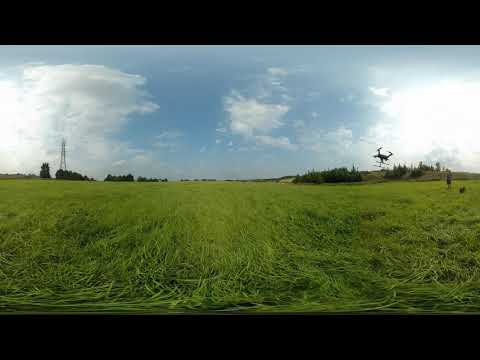This is a panoramic outdoor image captured with a fisheye lens, creating a slightly bent horizon. The scene is set in a large grassy field under the bright sunlight, hinting at the middle of the day. A prominent feature of the image is a large grassy field occupying the bottom half, with the upper half dominated by a gray but clearing sky filled with puffy white clouds. A solid black border frames the top and bottom of the image.

In the upper left corner, there's a power tower holding electrical lines. On the right side, just where the low sun is visible, a black DJI Phantom 3 drone with a four-rotor design and skids is seen taking off. Below the drone, there appears to be a person standing in the field. The grassy terrain shows rows of cut hay or grain, and a small island of pine trees can be spotted in the distance on the right. The colors in the image range from various shades of green for the grass, blue and white for the sky and clouds, to black and gray for the drone and the border. The setting is clearly outdoors, in a wide-open field under a partially cloudy sky.